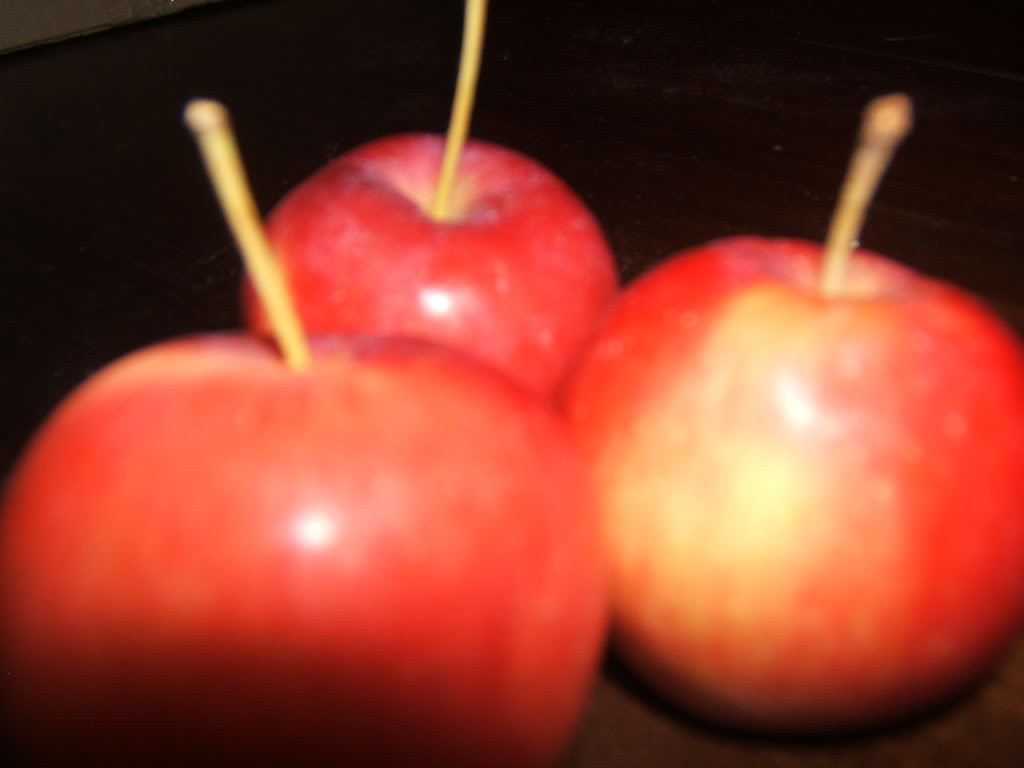This color photograph captures an extreme close-up of three red apples with a yellowish tinge. The apples dominate the frame, arranged in a triangular formation against a dark brown or black background, likely sitting on an indistinct dark surface. The lighting creates a glare, possibly from a camera flash, giving the apples an extra shiny appearance. Each apple has a long, straight yellow stem that appears slightly out of focus. The apple on the left is positioned closer to the forefront and is predominantly red with a yellow stem. Behind it, the apple on the left-back is solid red with a similar yellow stem. The apple on the right features a prominent golden patch on the front, standing out from the primarily red hue. Despite the overall image being blurry, the vivid colors and shiny surfaces are discernible. Small white specks can also be noticed on the apples, adding slight texture to their glossy surfaces.